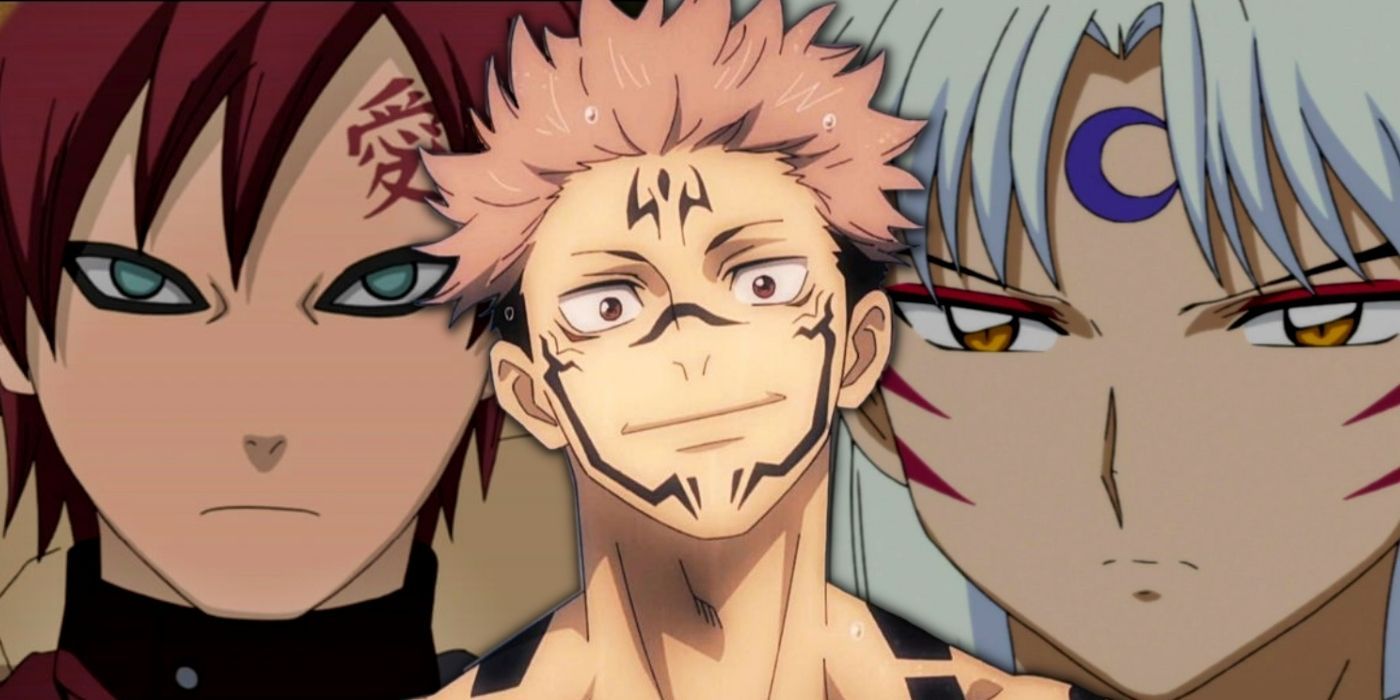The image depicts three prominent male anime characters, presumably from a widely popular series. Positioned centrally, the first character’s intense gaze and upper body are partially visible. His most distinctive feature is a burgundy Japanese tattoo decorating the side of his face. Flanking him on either side, the other two characters are shown in full profile. The character on the left boasts striking light brown hair and a black tribal tattoo intricately covering the top, middle, and lower portions of his face. Meanwhile, the character on the right has white hair, accentuated by a crescent moon tattoo prominently etched in the center of his forehead. Each character shares a serious, focused expression, adding to the intense atmosphere of the image. The varied hairstyles and unique facial tattoos add a layer of individuality to each character, making them distinct yet united in their determined demeanor.